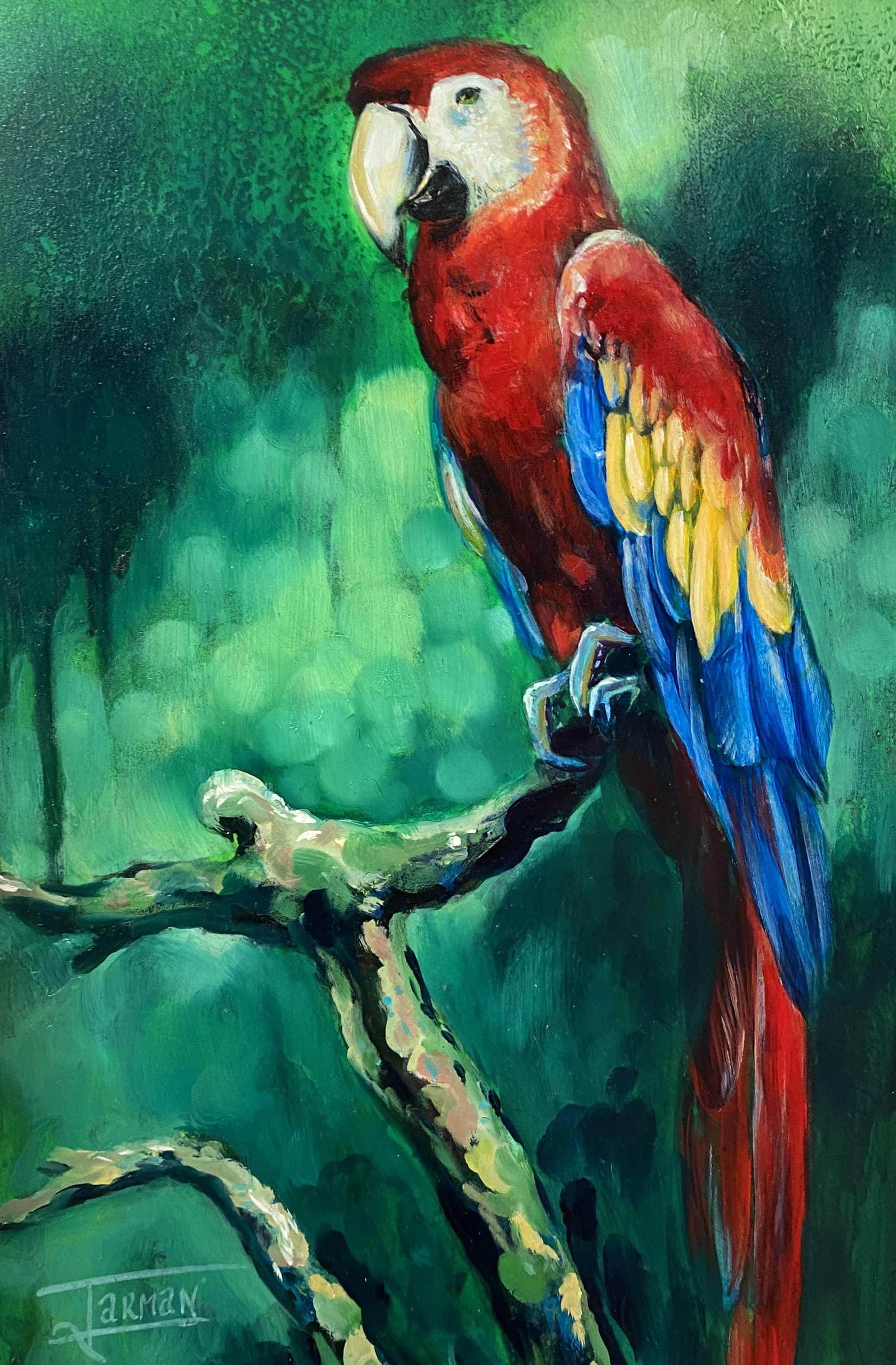This detailed painting captures a vividly colored parrot resembling the iconic toucan from the Froot Loops box. Showcased against a predominantly black and green background, the bird boasts a striking array of feathers: predominantly red on its body and tail, with blue tips on its wings, a patch of yellow on its mid-body and shoulder, and white around its eye and cheek. The parrot's green eye and neutral-colored, pointed beak are distinct features, as is the black marking under its beak. The bird is perched on a tree branch painted in shades of green and brown, extending from the bottom of the canvas. The artist's signature, "Jarman," is marked in the lower-left corner. The overall medium is oil on canvas, depicting an outdoor setting with hints of green trees interspersed with patches of black in the background. The parrot is positioned in profile, gazing towards the left side of the painting, with its head angled downward.